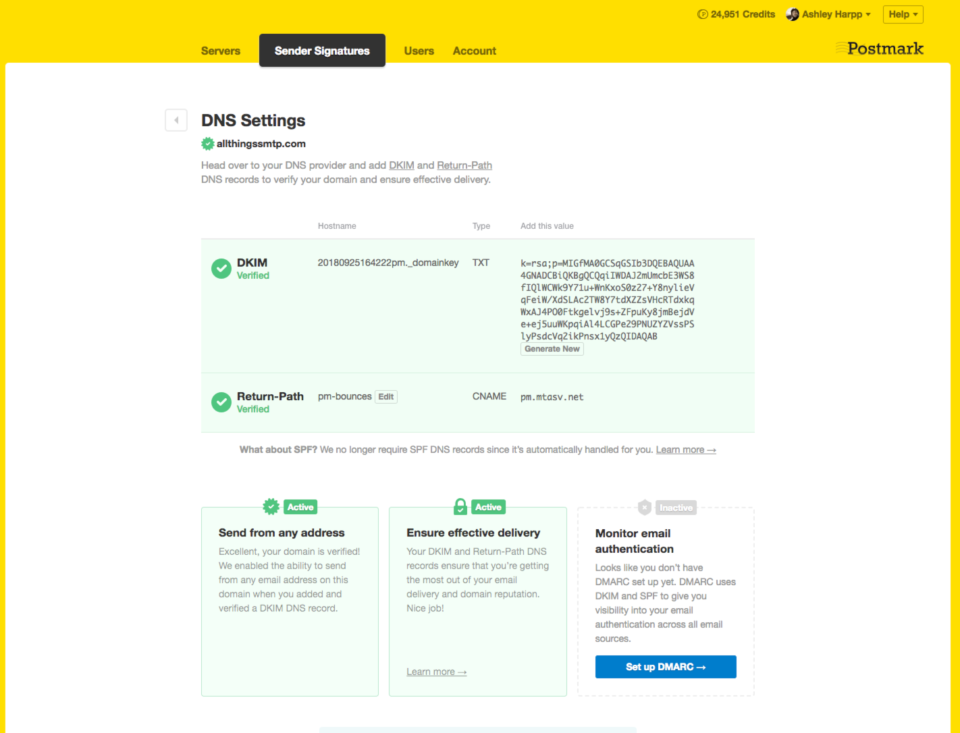The image depicts the settings menu of the Postmark platform, outlined in yellow and located in the upper right-hand corner. Prominently displayed at the top is the Postmark logo and brand name. Below the logo, a horizontal toolbar is visible, featuring tabs labeled "Servers," "Sender Signatures," "Users," and "Account." The "Sender Signatures" tab is currently highlighted in black, indicating it is the active section. Beneath this, the DNS settings are shown. Although the text within the DNS settings is too small to read, each setting is marked with a green circle containing a checkmark, suggesting that all existing DNS configurations are correctly set up. In the lower right-hand corner of the settings window, there is a section titled "Monitor Email Authentication," beneath which lies a prominent blue button labeled "Setup DMARC," ready to be clicked for further configuration.